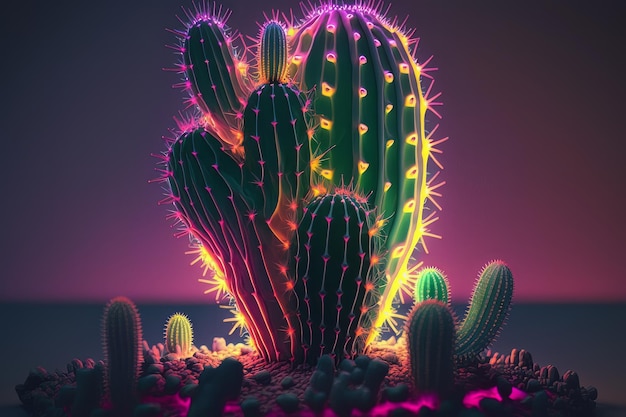A vivid artist's rendition showcases a group of cacti in a semi-realistic yet cartoony style. The central focus is a large, green cactus adorned with spines, radiantly backlit in neon hues of yellow and pink. Surrounding this dominant cactus are smaller cacti, also illuminated with vibrant pink and yellow light. The sharp contrasts in color create a striking effect against the blurred backdrop, which transitions from a dark upper third to a mix of purple and dark green lower sections. Detailed with a rock formation at the base, further cacti are scattered around, adding to the composition's complexity. The entire scene, from the glowing base to the neon-lit needles, exudes a sense of surreal vibrancy, highlighted even more by the sharp focus on the cacti against the muted background.